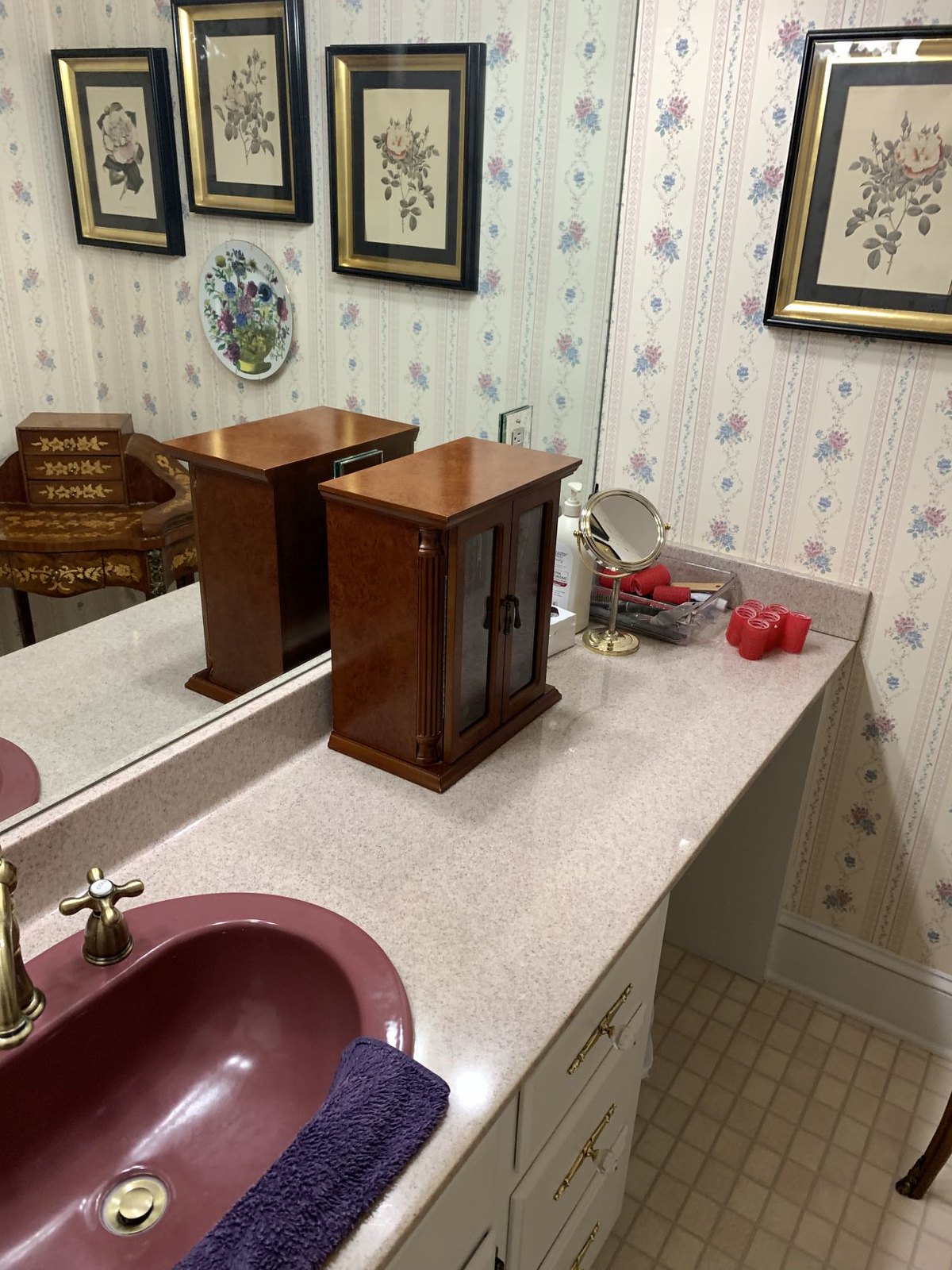The indoor bathroom photograph showcases a well-organized vanity area with an eye-catching mix of colors and textures. The shot captures the sink and vanity shelf, which extends the entire length of the left wall, featuring an open space beneath it where a vanity chair could be placed.

In the lower left corner, the oval sink stands out with its muted mauve-burgundy hue, accentuated by brushed brass fixtures. The entire left wall is adorned with a large mirror, enhancing the room's sense of space. Flanking the sink on the right, three white drawers add storage functionality.

The vanity countertop, adorned with a subtle peachy beige design on a white background, hosts a charming wooden jewelry chest with two glass doors, resembling a miniature piece of furniture. Adding a touch of elegance, a gold-toned stand mirror and several red hair curlers are also placed on the countertop.

The wallpaper features a vertically striped floral design in muted burgundy and pale blue, harmonizing with the sink's color and adding a vintage touch to the room. The flooring is a tasteful combination of white tile and pale grayish beige wood, enhancing the room's aesthetic. A chair's leg, visible in the lower right corner, hints at the potential comfort and usability of the space.